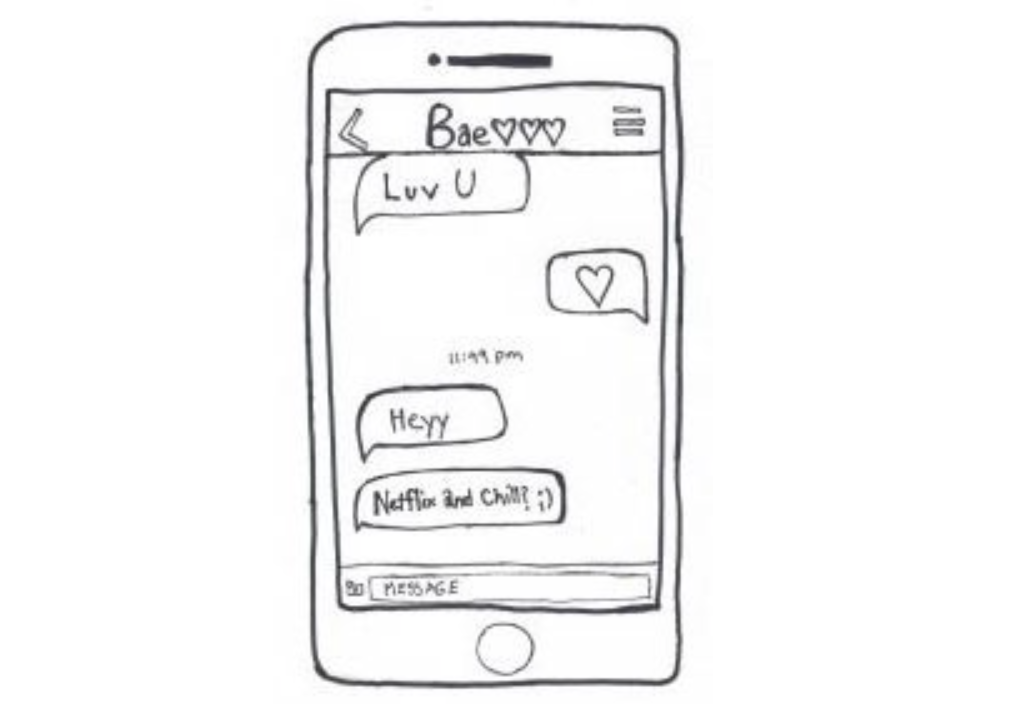This image is a black and white line drawing of an iPhone screen set against a white background. The drawing, done with a marker or pen, features a detailed depiction of a typical messaging app interface. At the top, the recipient’s name is shown as "BAE" with three heart symbols. The messaging sequence includes several casual, affectionate exchanges. The first message reads "LUV U" in a stylized word bubble, followed by a response that says "HEY" with an extra "Y" and a timestamp of 11:49 p.m. Below that, another message asks "Netflix and chill?" with a sideways wink emoji. The image concludes with a blank message bubble awaiting input and a drawing of a home button typical of iPhone screens. The artwork focuses on capturing the intimate and playful nature of text messaging between partners, emphasizing the theme of love and connection.